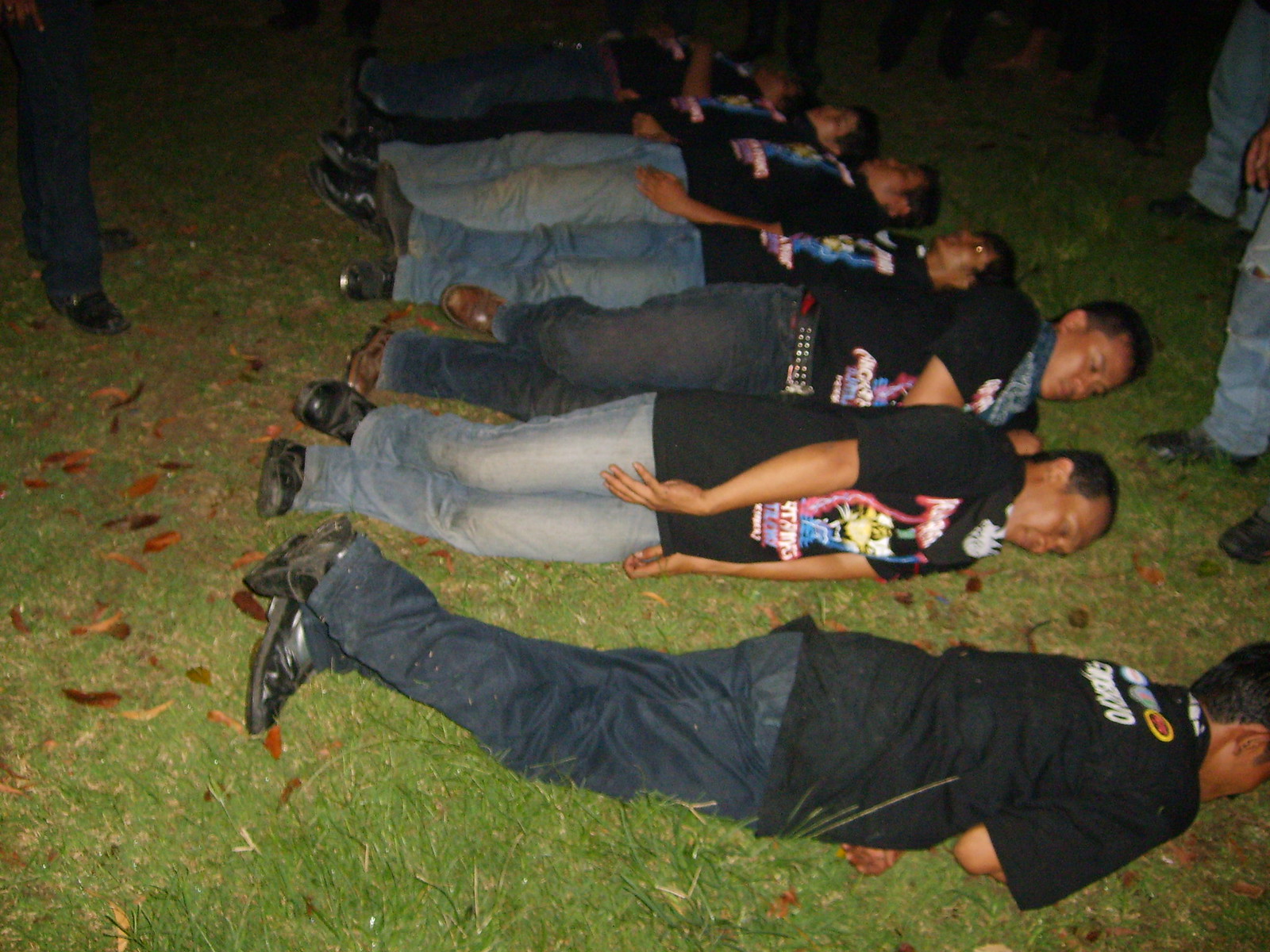This photograph showcases a group of young men dressed in dark shirts, mostly black, and blue or dark jeans with black shoes, sprawled out on a grassy area with scattered brown leaves. Most of the men are lying horizontally on the ground in various positions—face down, on their sides, or on their backs—giving an impression of either playfulness or exhaustion. The scene is captured at night, adding a shadowy, mysterious quality to the image. Around them, other individuals stand, observing with amused expressions, suggesting a communal activity or initiation possibly linked to a college group. The contrast of green grass and brown leaves, combined with the somber clothing of the men, adds texture and depth to the image, emphasizing the camaraderie and lightheartedness of the moment despite the seemingly chaotic scene.